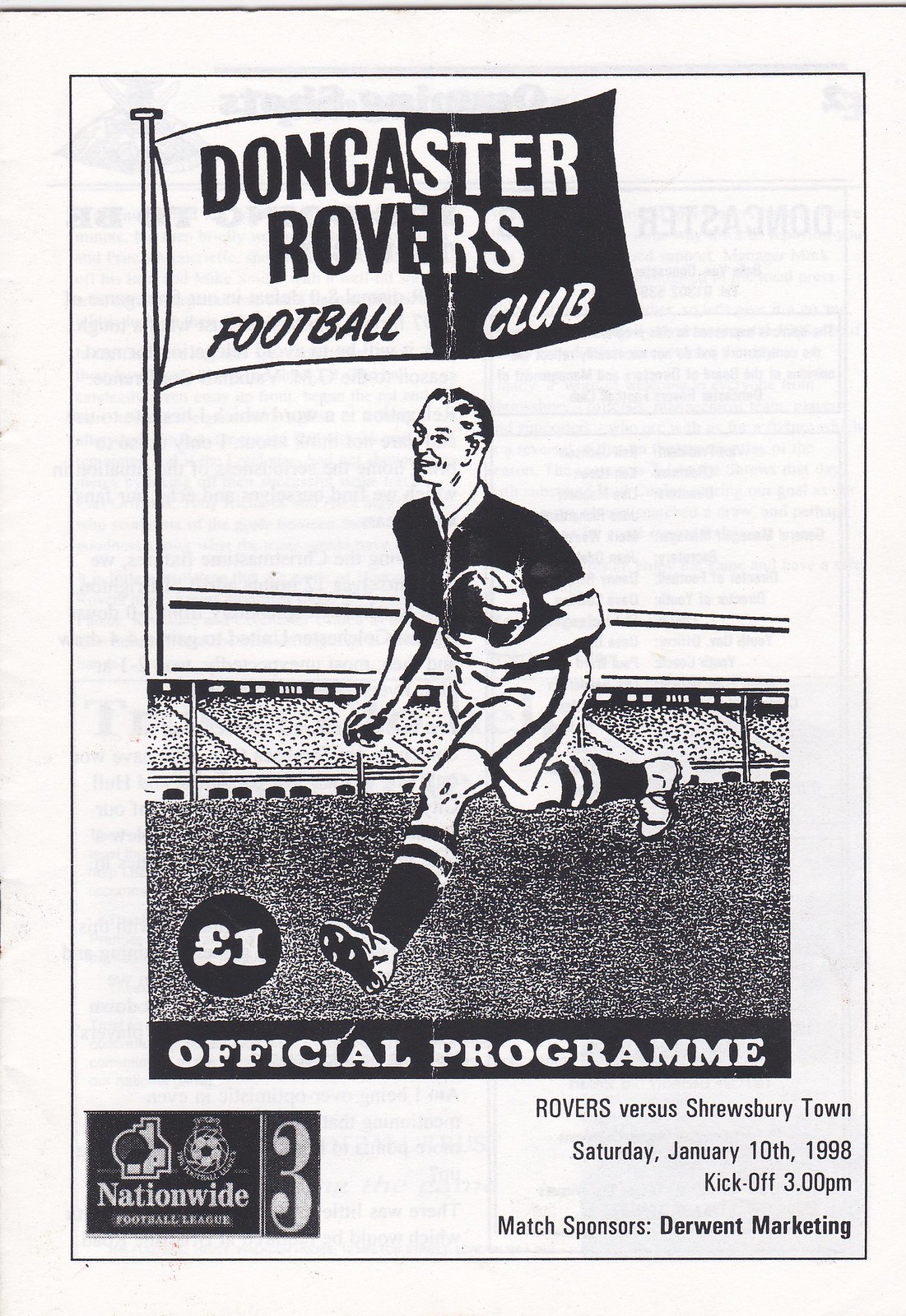This black and white image is a vintage advertisement, likely from a magazine or newspaper, featuring a Doncaster Rovers Football Club match program. At the top, a two-toned flag with "Doncaster Rovers Football Club" marks the club's identity. Below this, an illustration shows a man running down a field with a soccer ball, dressed in a black jersey with white trim on the sleeves and collar, white shorts with a black stripe, and black socks with two white stripes. In the background, stands are filled with spectators. The text below the illustration reads, "Official Program, One Euro." In the lower right, details of the match are provided: "Rovers vs. Shrewsbury Town, Saturday, January 10, 1998, Kickoff 3 PM. Match Sponsors, Derwent Marketing." The lower left also mentions, "Nationwide Football League, Three," with a realistic logo. The background, made of very thin paper, reveals text from the reverse side.